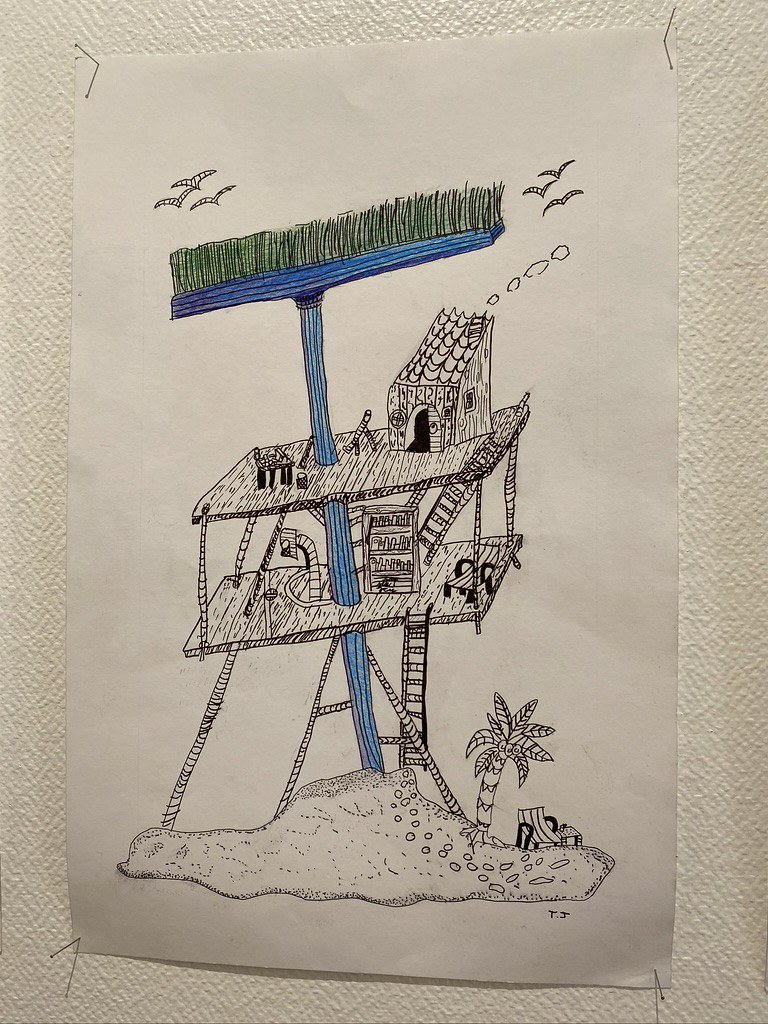Captured in this image is a rough-textured white wall, emphasizing its coarse, uneven surface. Affixed to the wall at all four corners is a sheet of white sketch paper, displaying a vibrantly colored marker drawing. The illustration depicts a serene island scene, with a prominent palm tree positioned on the right side, beneath which a solitary chair rests, inviting relaxation. Intriguingly, the scene features a blue broom with green bristles, positioned upside down and protruding from the sand. This broom forms part of an imaginative structure with multiple floors: connected by a series of ladders, two floors lie beneath the broom, ultimately leading up to a house perched at the apex of this whimsical tower.